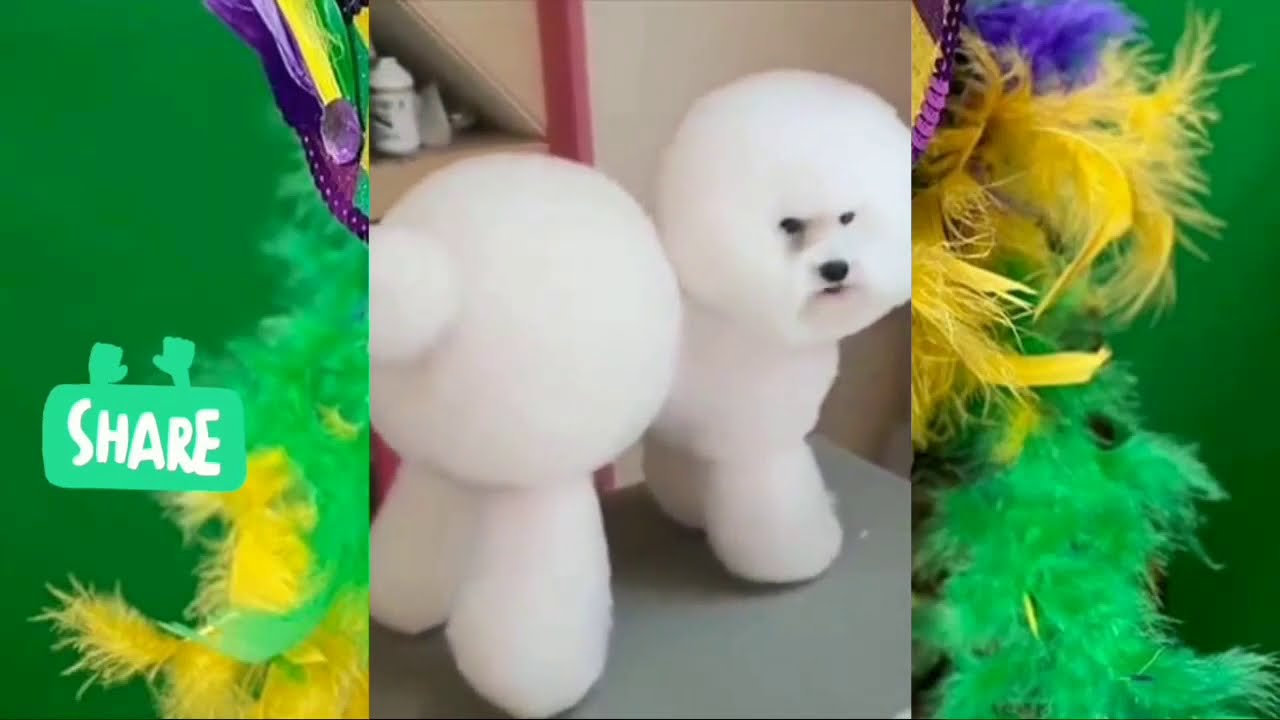The image is a horizontal rectangular picture split into three vertical panels. The central panel prominently features a poodle that appears so meticulously groomed it almost resembles a figure sculpted from styrofoam. The poodle boasts a strikingly circular head, body, and tail, with realistic black eyes and nose, standing on a gray platform or countertop against a white wall with some red trim. The left and right panels showcase a vividly colorful background dominated by darker green hues. On the left panel, the background is adorned with green, yellow, and purple feathers at the top and bottom, and includes bold white text that reads "SHARE." The right panel mirrors this with similar feathers in varying shades of green, yellow, blue, and purple. The overall contrast between the fluffy white poodle and the vibrant, feathered panels creates a unique and engaging visual.